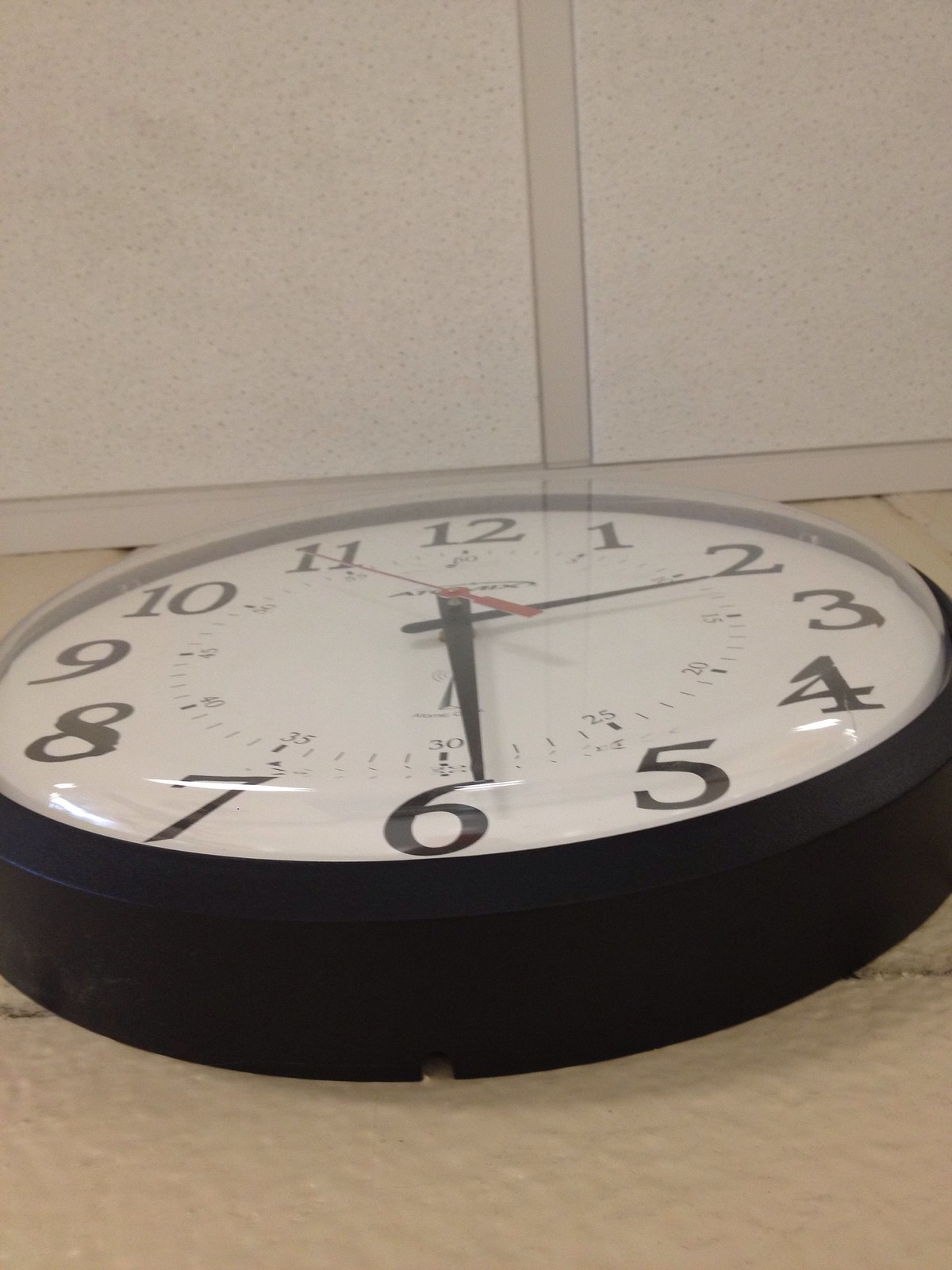Caption: 

The image captures a partial view of a round wall clock mounted on a light-colored stone surface. The stone background has visible indentations, suggesting it was used as masonry with adhesive for stacking bricks. The surface is textured and bumpy, resembling traditional brickwork. Above the clock is a cream-colored, paneled ceiling typical of institutional or commercial spaces. The clock itself features a black plastic frame and a transparent bubble-style cover. Inside, it has bold black numbers and black hour and minute hands, accompanied by a vibrant red second hand, all set against a stark white background. Parts of the clock are cropped out at both the left and right edges of the image.